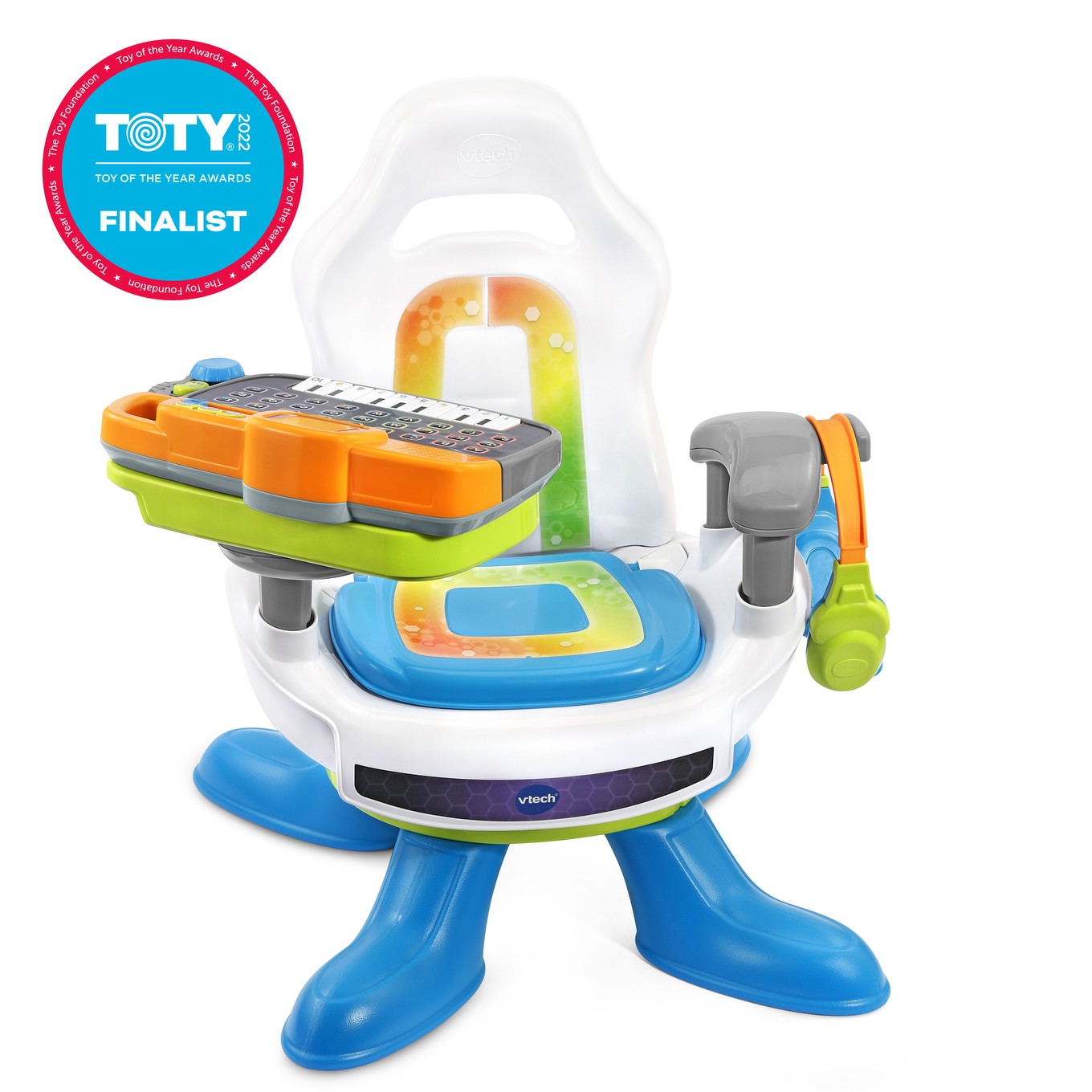In the image, we're looking at a detailed depiction of a children's toy, likely manufactured by VTech, photographed against a completely blank white background. The central object is a computer-like chair, predominantly white with four blue legs. The seat has a unique, colorful design featuring a mix of orange, yellow, and green around its inner perimeter, transitioning into a solid blue middle section. The chair is equipped with two gray armrests. Hanging from the armrest on the right side of the image (left side of the chair) are a pair of distinctive headphones, with an orange top, a green cup on the left headphone, and a blue cup on the right headphone. On the opposite armrest (left side of the image, right side of the chair), there is an orange and green keyboard that appears to have both piano keys and letter buttons, indicating multifunctionality. The toy appears to be made entirely of plastic. Additionally, in the top-left corner of the image, there is a blue circular badge surrounded by a red outline, with white text indicating "TOTY 2022 Toy of the Year Awards Finalist," highlighting the toy's accolade.